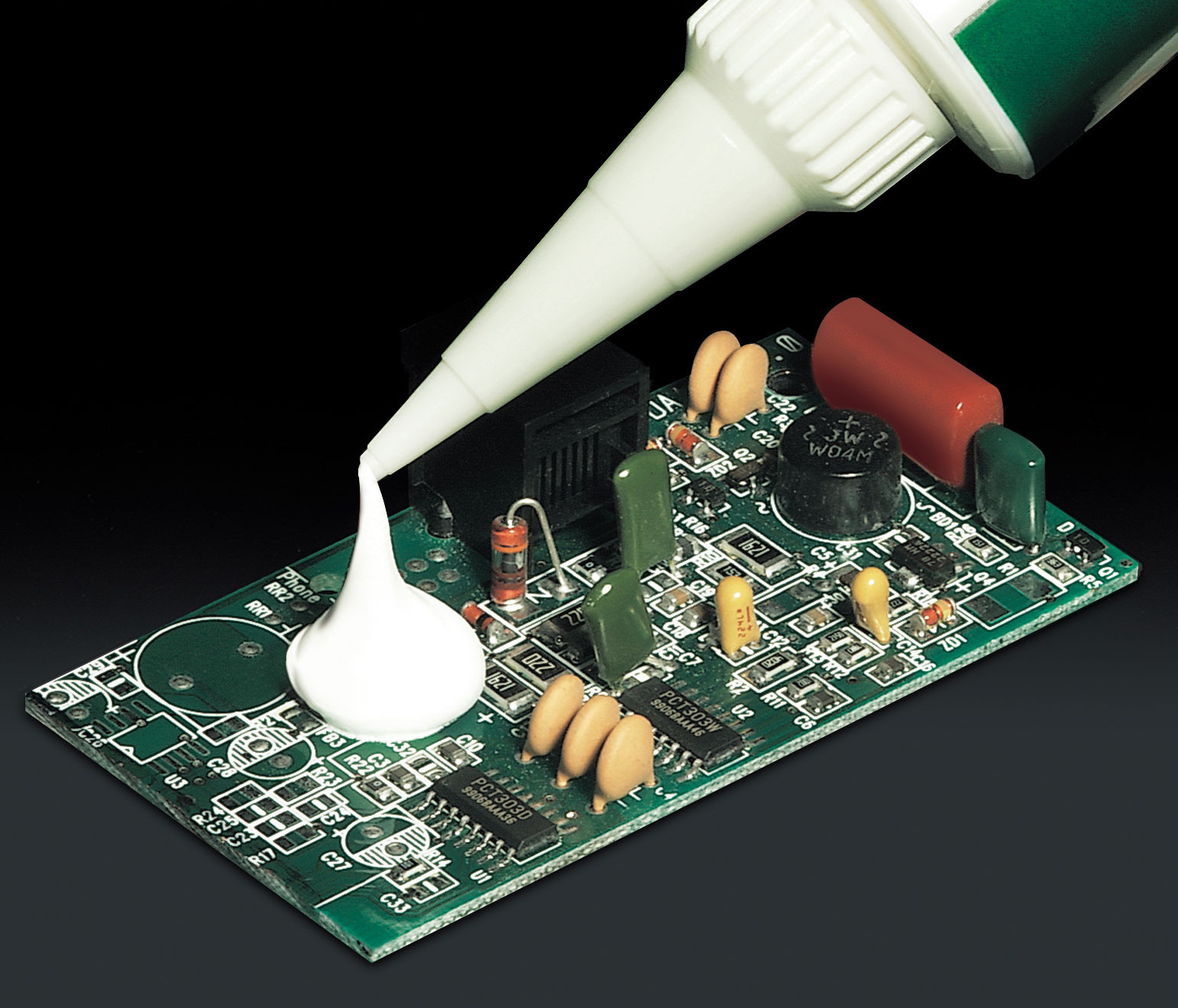This detailed photo captures a close-up view of a green circuit board or motherboard, set against a black background. The board is densely populated with various components, including white rectangles and lettering, small tan and red batteries, as well as numerous circuits and electrical inputs. There's a distinctive white outline encasing the entire module. Prominently, from the top right corner, a large bottle is dispensing a sizable dollop of white glue onto the left side of the circuit board. The glue, appearing almost quarter-sized, contrasts starkly with the meticulous, intricate components of the board, lending a nonsensical and potentially destructive quality to the image.